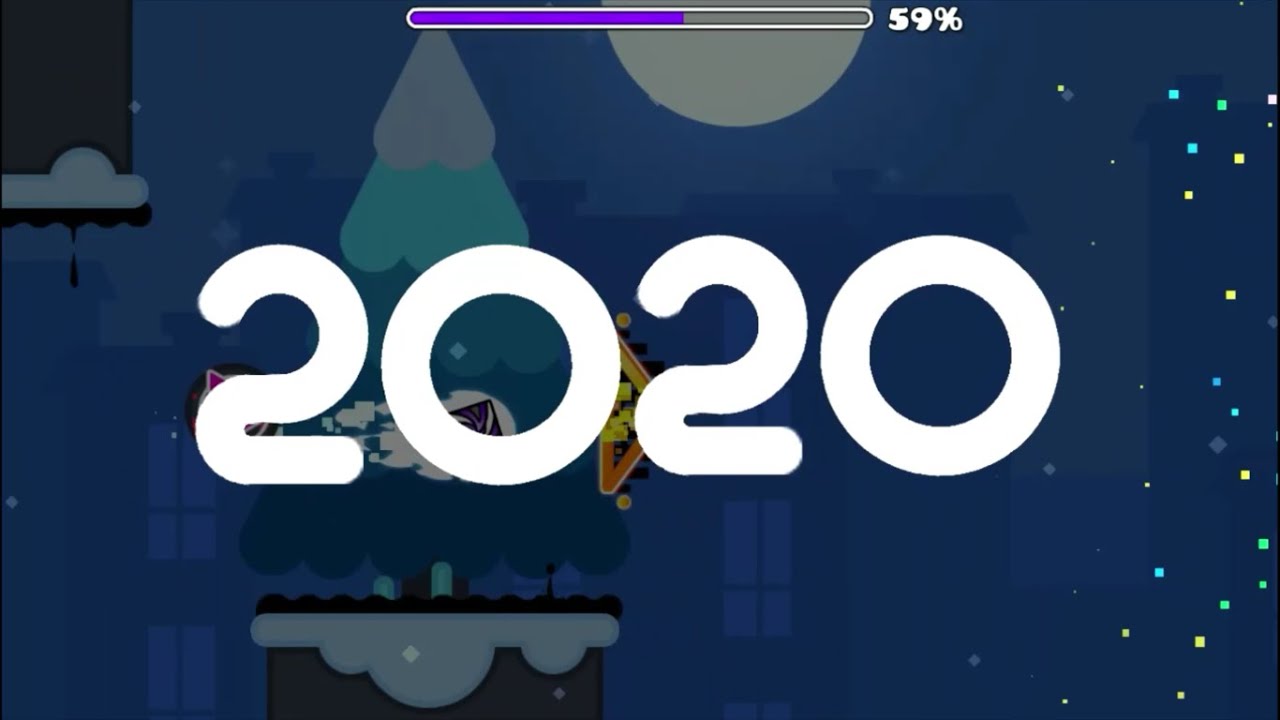A partially loaded screen capture from a video or animated GIF, showing 59% completed. The focal point is a large "2020" written in rounded letters or numbers, set against a minimalist design reminiscent of Minecraft. A snow-covered tree stands prominently in the scene, its simplistic and blocky design adding to the pixelated aesthetic. Positioned in the center of the image is a play button, indicating that this is, indeed, a video. To the right of the tree, sparkling dots, likely representing stars, are visible, enhancing the nighttime ambiance. In the background, a full moon glows brightly, completing the tranquil wintry setting, suggesting this might be a New Year's video celebrating the advent of 2020.